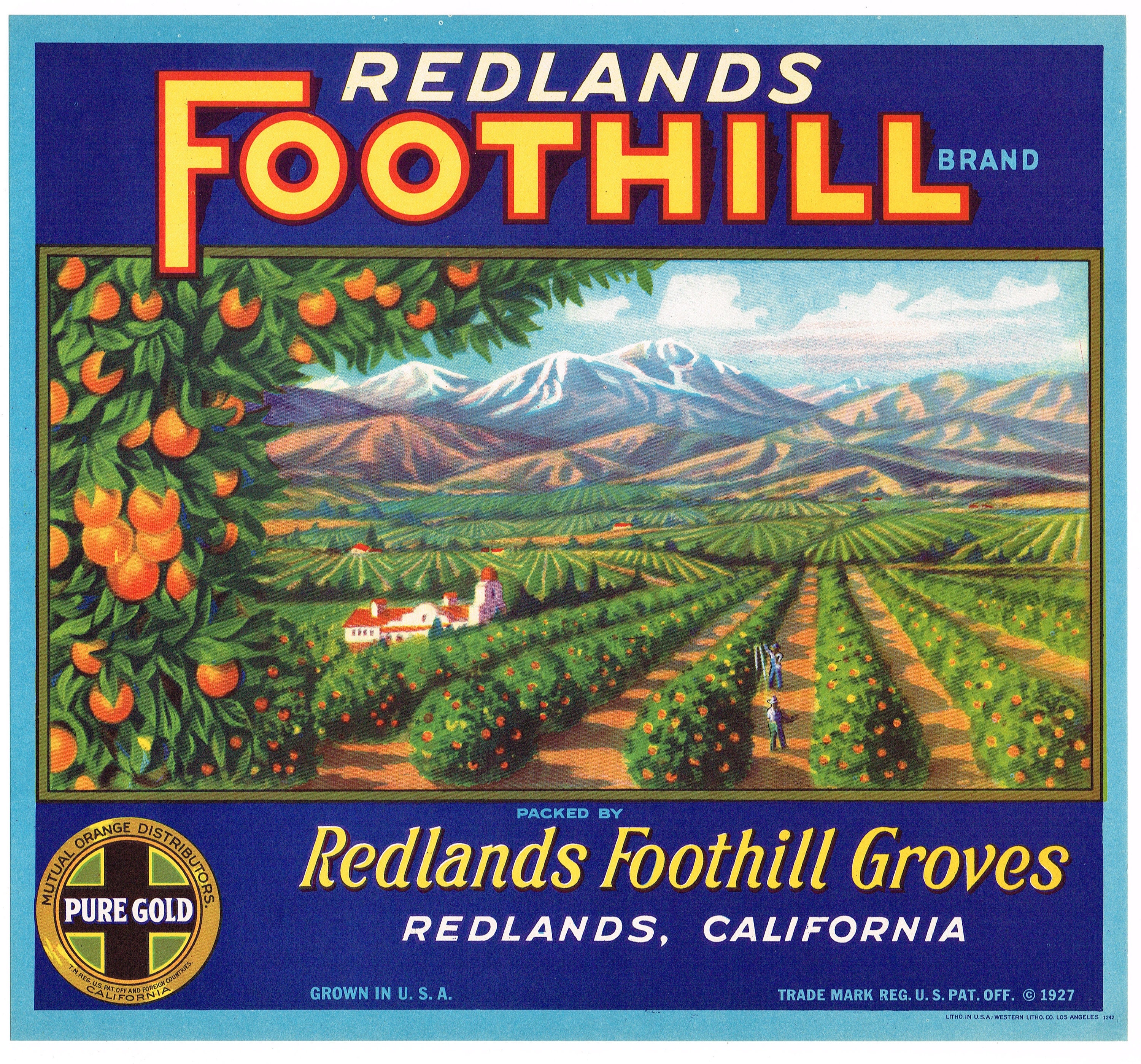This is a detailed digital poster advertising Redlands Foothill, a distinguished brand of oranges, set against a picturesque backdrop. The poster features a light blue border with dark blue bands at the top and bottom. The top band prominently displays "Redlands" in a light cream font, followed by "Foothill" in yellow with red outlines, and "Brand" in blue to the right. The central illustration vividly depicts rows upon rows of orange trees, laden with vibrant oranges against brown soil, extending into the distance. Harvesters are shown picking the ripe fruits. To the left, a closer depiction of an orange tree adds depth. The landscape in the distance features low-lying hills and majestic snow-capped mountains beneath a bright blue sky dotted with white clouds. At the bottom of the poster, the text reads "Redlands Foothill Groves, Redlands, California" in a yellow font, complemented by a "Pure Gold" seal, and "Grown in the USA" to emphasize the origin. A small white house can be spotted on the left, adding a touch of cozy rural charm. The design is completed with a mention of '1927' at the bottom, enriching the heritage aesthetics of the label.